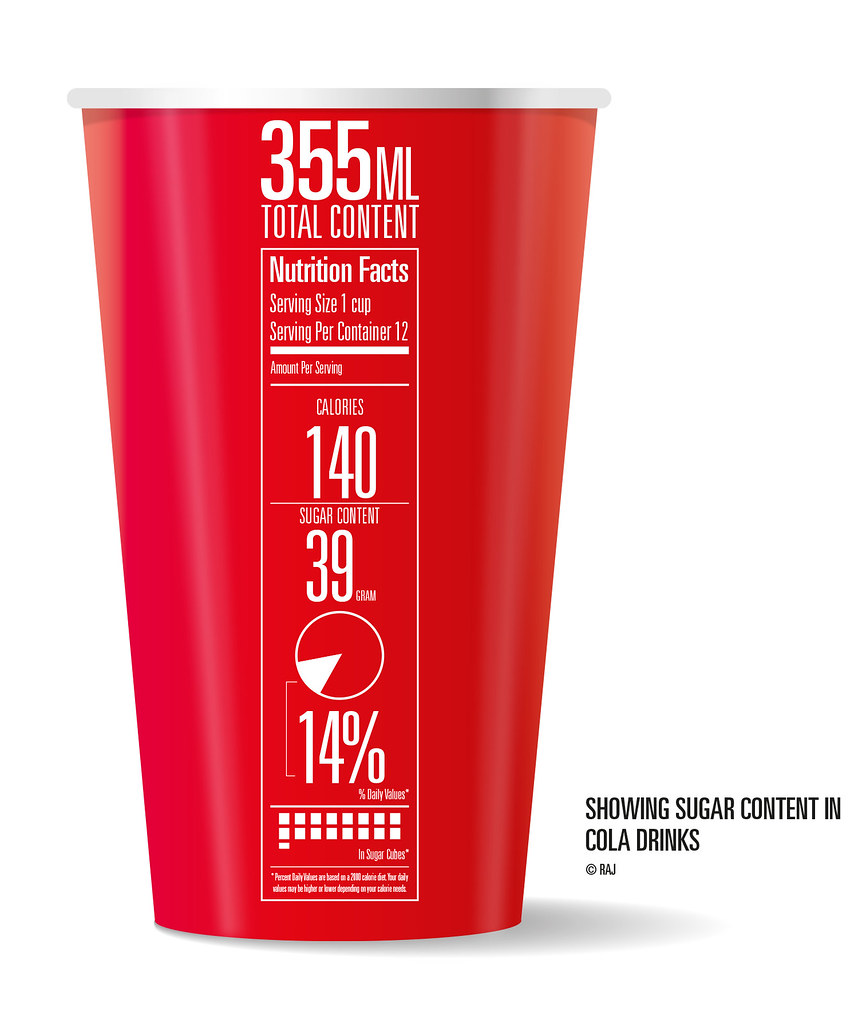This detailed infographic illustration features a tall red paper cup, similar in shape and style to those used in restaurants for dispensing soft drinks. The cup displays several white graphics, beginning with a text that specifies the total content: 355 milliliters. Following this, a comprehensive nutrition facts segment indicates that the serving size is one cup, and each container holds 12 servings. Furthermore, it details that each serving contains 140 calories and 39 grams of sugar, which amount to 14% of the recommended daily value for sugar.

The nutritional information is organized in a format reminiscent of standard nutrition labels, making it easy to read. Below these details, a pie chart visually represents the 14% daily value for sugar intake. Complementing the pie chart, a pictograph displays the equivalent sugar content in the form of sugar cubes, totaling 16 and a half cubes. This visual aid starkly illustrates the high sugar content. 

On the right side of the infographic, set against a white background, black text states, "Showing sugar content in cola drinks," along with a copyright mark for RAJ. The cup itself features a reflective, waxy appearance with a rolled white rim, further enhancing the realistic presentation of the paper cup.